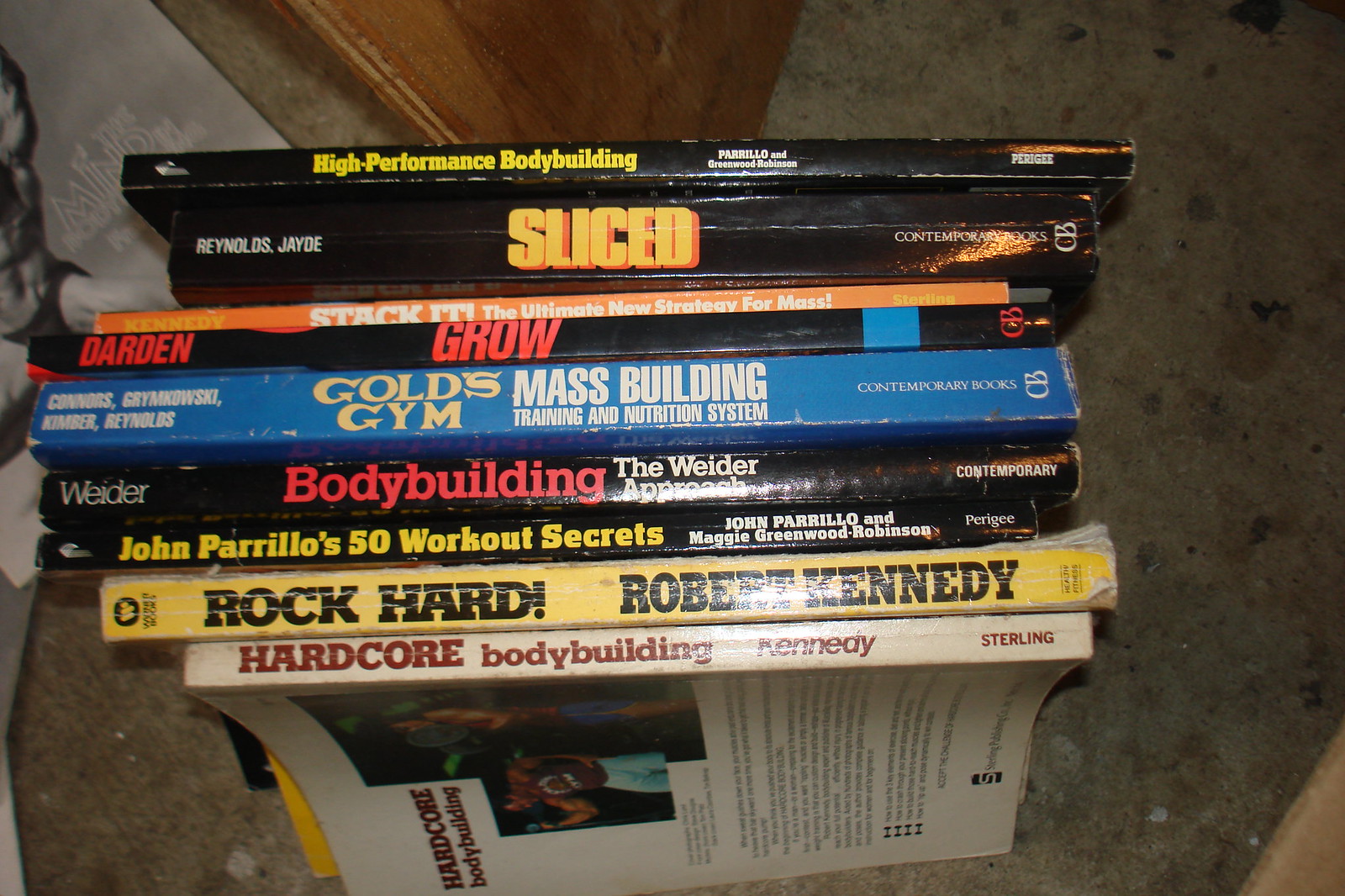The photograph captures the spines of ten bodybuilding-themed paperback books arranged vertically, propped up on their pages within an indoor setting. They rest on a grey, older-style concrete floor that is visible in the corners and speckled with black and brown stones. In the upper left corner of the image, a white object with the text "The Mind" in bubble print is slightly visible. The book titles and their descriptions are as follows:

1. **High Performance Bodybuilding** - Black cover with yellow font.
2. **Sliced** by Jade Reynolds - Black cover with white font.
3. **Stack It: The Ultimate New Strategy for Mass** - Thin, orange cover with white font.
4. **Grow** by Ellington Darden - Black cover with white font.
5. **Gold's Gym** - Thick, blue cover with gold lettering, underneath it reads **Mass Building Through Training and Nutrition** in white.
6. **Bodybuilding: The Weider Approach** by Joe Weider - Black cover with red title and white subtitle.
7. **John Perillo's 50 Workout Secrets** by John Perillo and Maggie Greenwood Robinson - Black cover with yellow-gold and white text.
8. **Rock Hard** by Robert Kennedy - Yellow cover with black, bold font.
9. **Hardcore Bodybuilding** by Robert Kennedy - White cover with red font.

This detailed arrangement highlights the various aspects of the books, including their titles, colors, and authors, set against the distinctive concrete flooring.